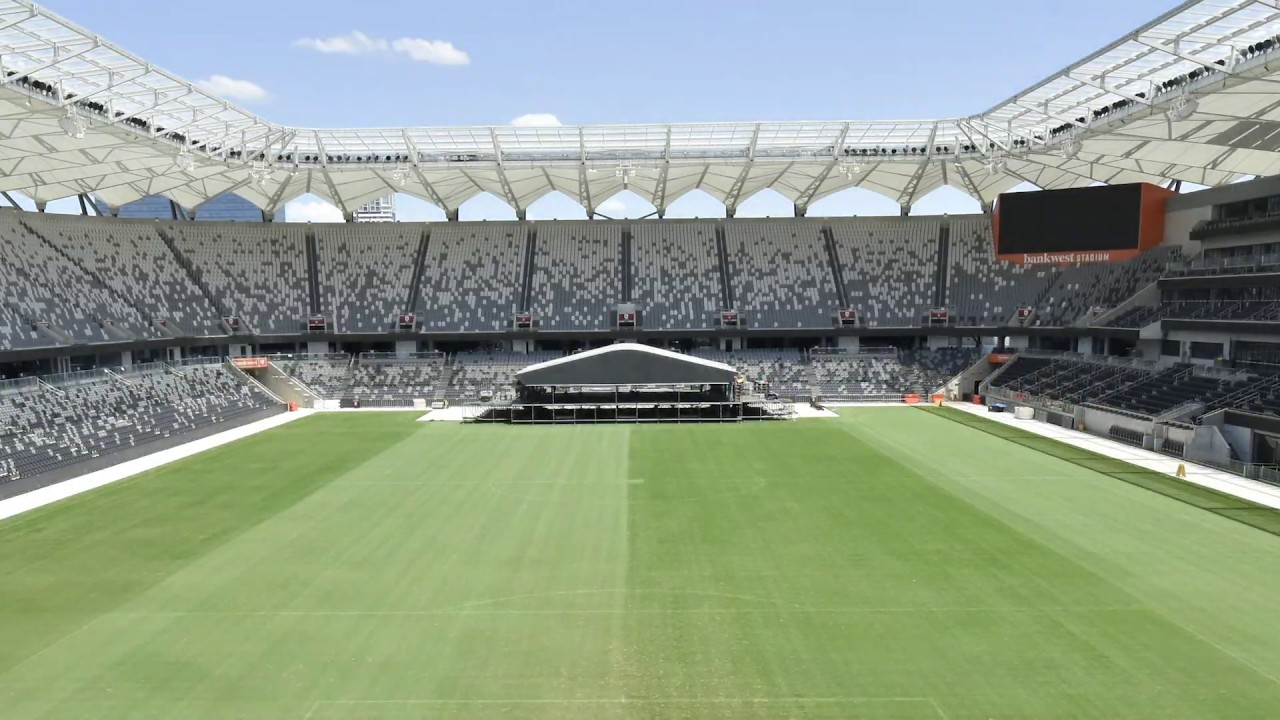The image depicts a detailed artist's rendering of Bank West Stadium, showcasing a vibrant and dynamic scene within a partially open, architecturally impressive structure. The stadium boasts a lush green grass field, bordered by a distinctive white awning that provides shade for the vacant bleacher seats, which create a striking speckled pattern of white and gray. A black scoreboard with a bold red trim sits on the right-hand side, displaying the stadium's name. At one end of the field, a large, covered stage structure stands prominently, suggesting preparations for an upcoming concert rather than a sporting event. The sky above is clear blue, dotted with large white clouds, adding a serene backdrop to the bustling preparations below. The field itself is faintly marked with the lines of a soccer pitch, and a sizable gray and white canopy, approximately 20 feet by 40 feet, is set up on the field, emphasizing the non-sporting use of the space for the time being.